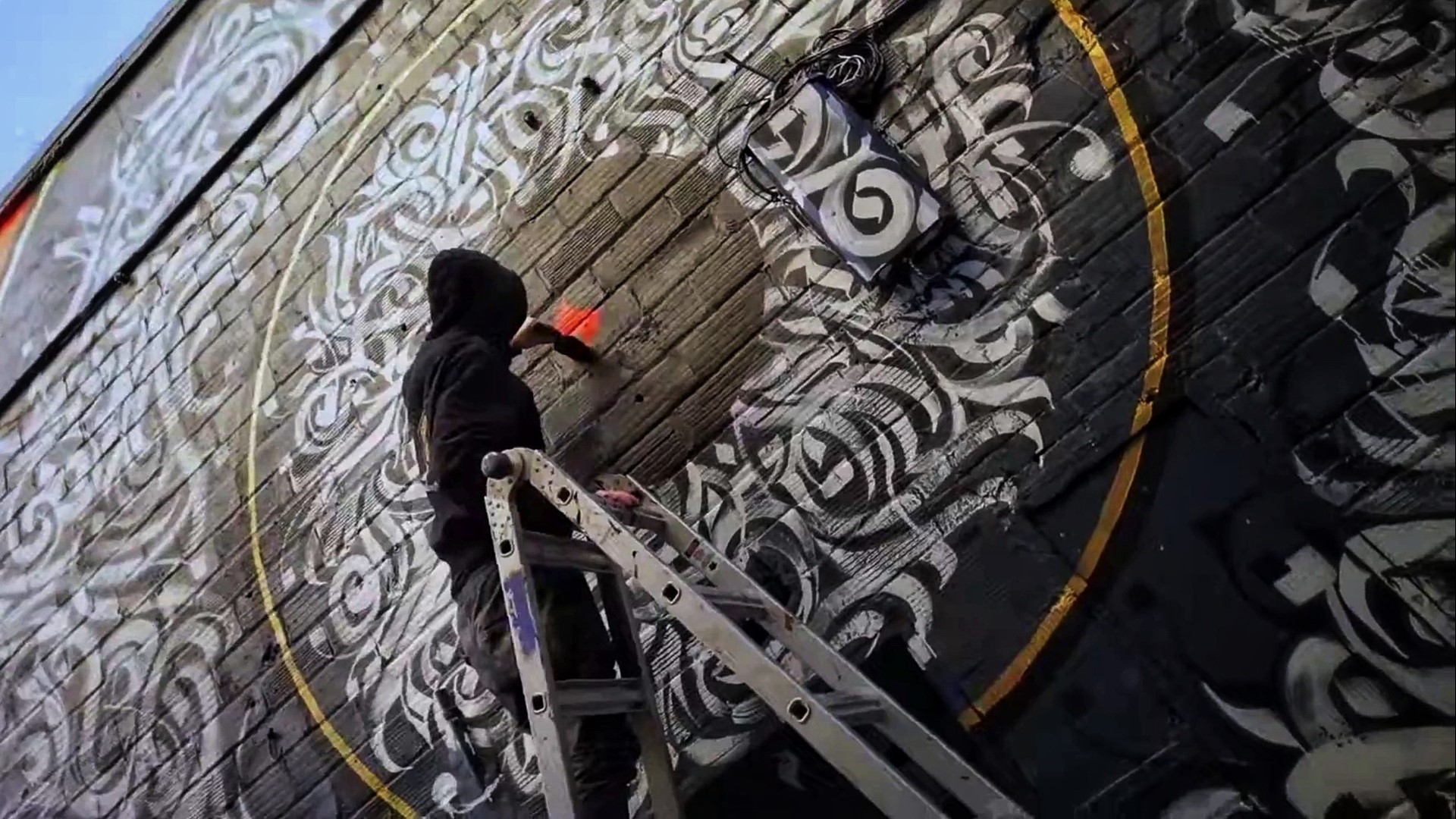In this outdoor daytime photograph, a person stands on a chrome ladder with a smudge of purple paint on its left side. The individual, whose back faces the viewer, is attired in a black hoodie with the hood up and dark, baggy pants. They appear to be painting an intricate design on the side of a structure constructed of dark brown, rectangular blocks, resembling either wood or brick. The sky in the top left corner is clear and blue.

Central to the artwork is an orange circular line, framing a complex pattern of white curves and lines that together form a tribal-like circle. Within this, a section of the design contains another orange element that seems to be the focus of the person's painting efforts. Surrounding the central motif is an additional layer of matching white curls and swirls, creating a donut shape. This design radiates outwards, contributing to an overall aesthetic that is detailed and elaborate, reminiscent of calligraphy.